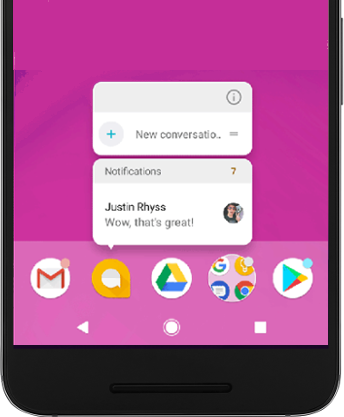In this image, the background is a vivid purple, framed by black outlines on the left, right, and bottom edges. Central to the image is a light gray area featuring an eye icon within a gray circle. Directly beneath this eye icon, there is a blue plus symbol encased in another gray circle. Below this section, partially visible text reads "New Conversation," which is truncated and followed by two horizontal lines.

In the next section, outlined in gray, the text "Notifications" is displayed with the number 7 placed to the right. Underneath this notification header, the name "Justin Rice" appears along with the text "Wow, that's great," accompanied by a small profile image of a person on the right side.

Further down, there's a series of icons representing different applications or services. The first icon shows what looks like a white circle with a red "M," likely representing Microsoft. Following this, the next icon features an orange border around a white circle. Adjacent to it is another white circle containing a multicolored triangle in yellow, green, and blue. The subsequent icon is Google's Chrome logo, characterized by a circular shape with segments in orange (right), blue (bottom left), and white (top left). Next, there’s a blue, red, and yellow triangle along with a blue circle containing a blue dot in the center.

In the bottommost section, there are three symbols: a white arrow pointing to the left, a white circle in the middle, and a white square on the right side.